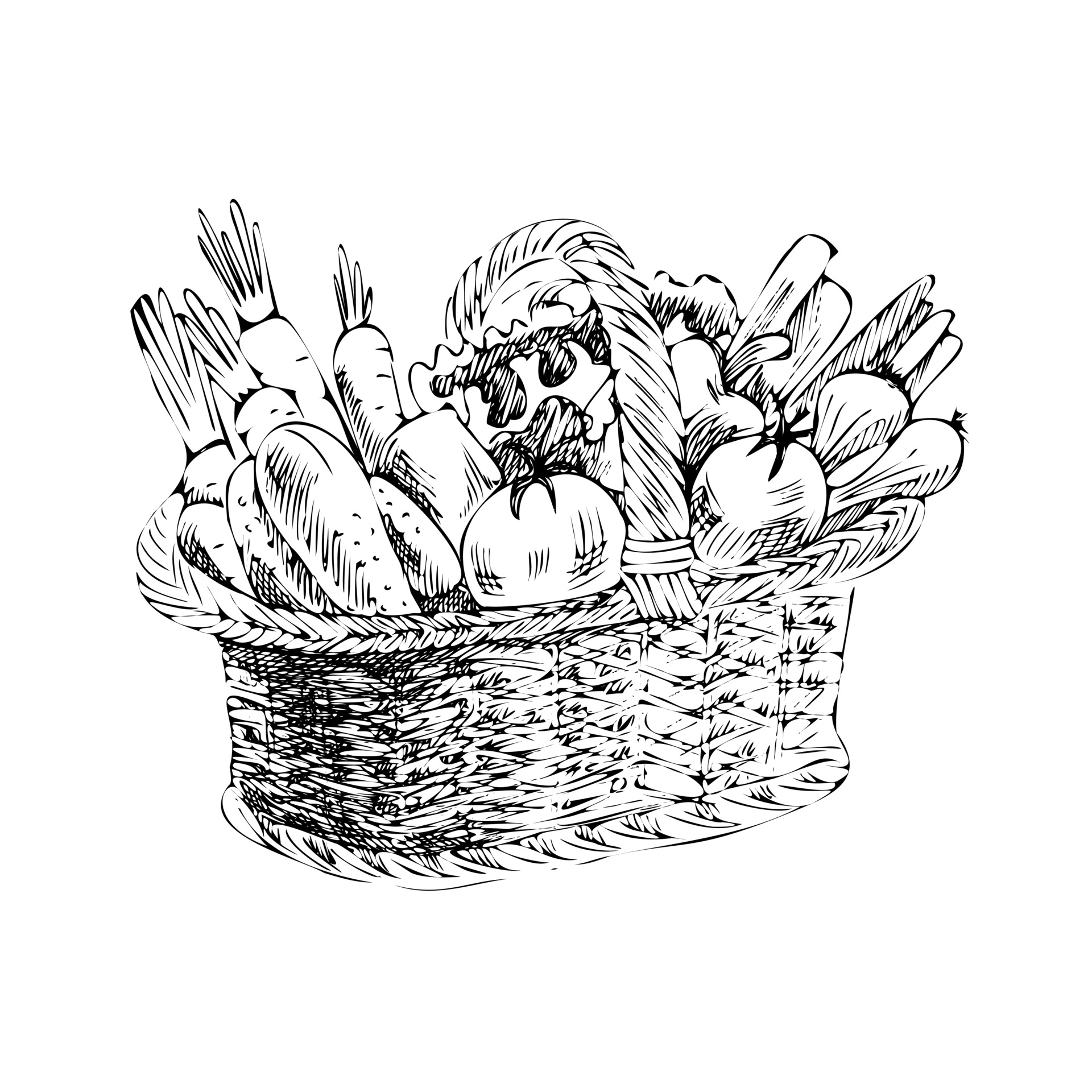An intricate fine line pen drawing on a white background, rendered in black ink, depicts an overflowing wicker basket filled with various produce. The oval-shaped basket, turned slightly to the right, features a central handle and is meticulously detailed, showcasing thicker, darker, and scratchier lines on the left side to suggest shadow, with more light on the right. The basket brims with an abundant assortment of vegetables that includes prominently placed carrots, tomatoes, leafy lettuce or cabbage, peppers, and potentially parsnips, arranged in such a way that the basket appears unable to accommodate any additional produce without spilling.